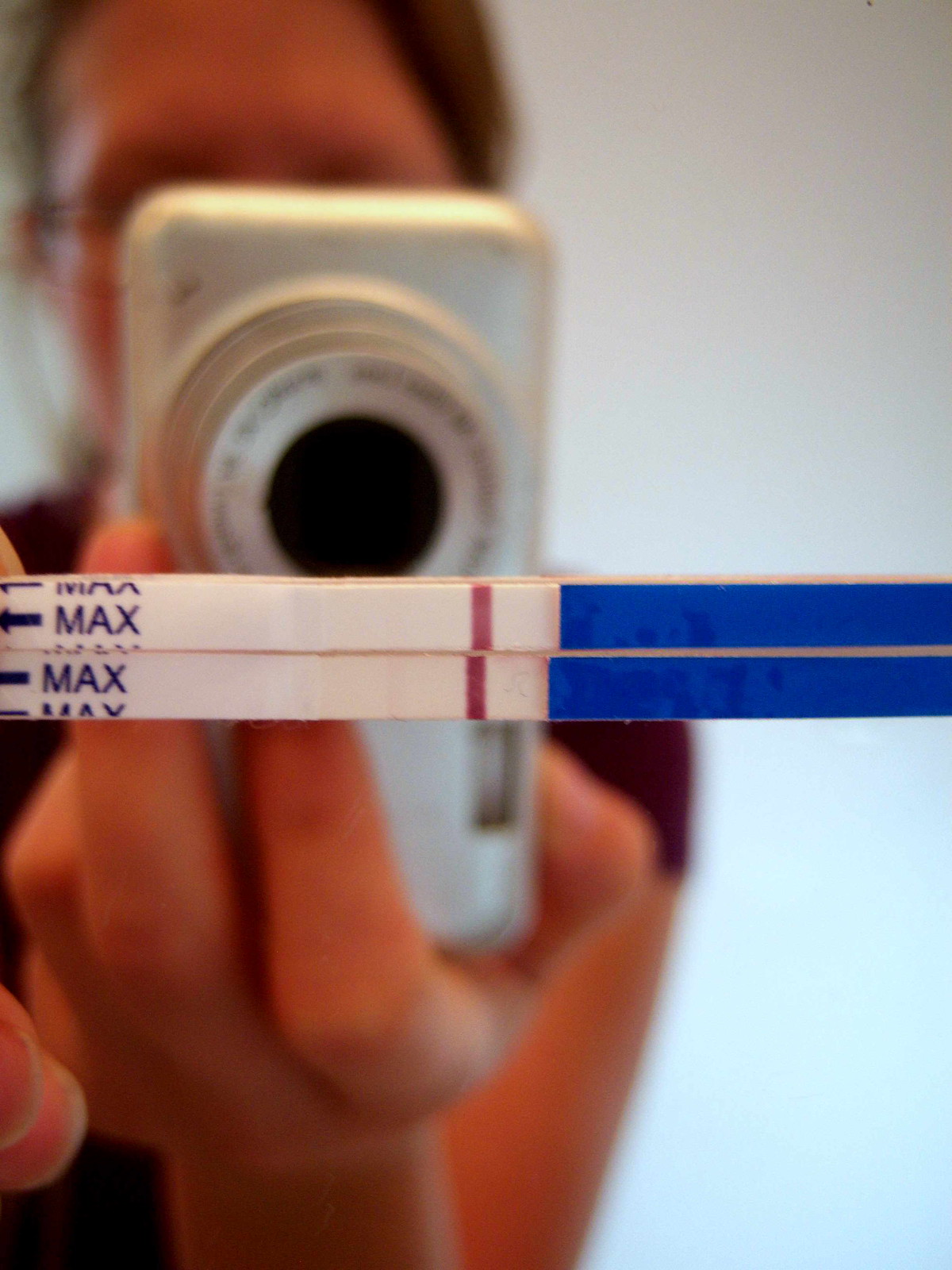In this highly blurred image, the focal point appears to be a Caucasian individual with noticeably red skin. Positioned towards the top left corner, this person sports brown hair on either side of their head and is presumably wearing glasses. Their dark eyebrows are faintly visible. 

Central to the image is a silver camera, identifiable by its conspicuous round lens, black at the center, and surrounded by three adjustable, elevated rings. Illegible writing is observed on the outermost silver ring. 

Dominating the middle of the picture are two horizontal bars. At the far left, the word "Max" is repeated in dark blue, interspersed with blue arrows pointing left. This pattern sits on a white strip, followed by a thin vertical red strip, another white section, and a bright blue strip. 

Below these bars, part of the camera’s body is visible, held by the person's left hand. The individual is dressed in a burgundy short-sleeved shirt, with the upper arm and fingers distinctly visible as they grip the camera. A mysterious red or light pink element is seen just below the hand, adding an additional layer of ambiguity to the scene.